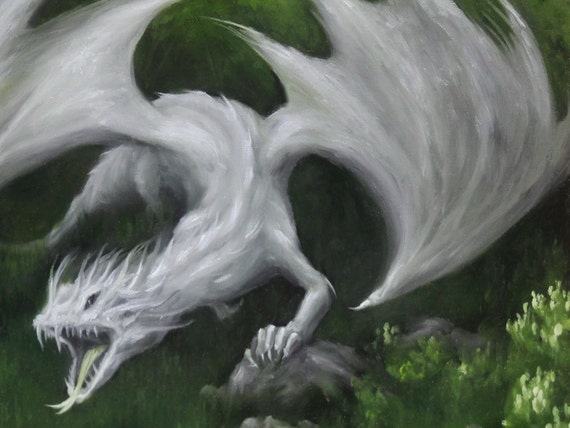This digital artwork presents a striking depiction of a dragon, positioned prominently at the center of the composition. The dragon's body is a pristine white, accentuated by an enormous, elongated green tongue that protrudes from its completely black mouth. Its small eyes emphasize the sheer size of its wings, which are about seven times the size of its head. The dragon's ferocious roar exposes its large fangs as it leans forward, grasping a gray rock with one extended clawed hand. Its imposing wings, stretching wide from its back, add to its formidable presence. The dragon stands amidst a sparse field of poorly defined green grass, interspersed with wildflowers on the bottom right, their bright hues providing a stark contrast to the predominantly dark, moody background of black and dark green shades. The entire scene captures the moment's tension, as if the dragon is either ready to breathe fire or is in a state of powerful outcry.